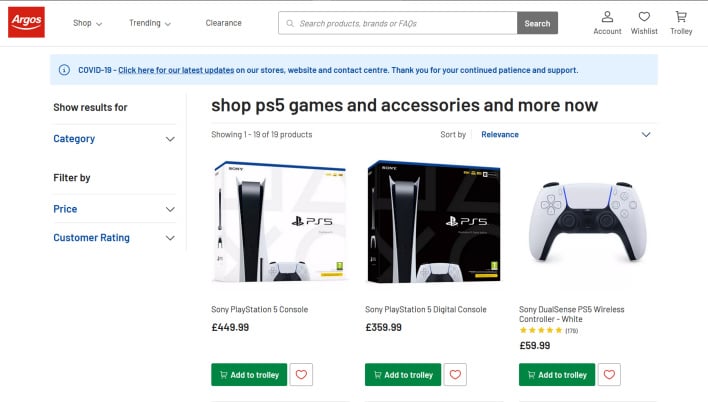The image is a horizontally rectangular frame showcasing a page from Argos' website with a primarily white background. At the top of the page, the recognizable red Argos logo is positioned in the upper left corner. To the right within the same banner, a navigation menu is displayed, consisting of the options: "Shop" and "Trending," both featuring drop-down arrows. Following these are the "Clearance" section, the search field, and on the far right, icons for "Account," "Wish List," and "Trolley," the latter symbolizing the shopping cart icon.

Directly beneath this main banner, there is a light blue horizontal bar with dark blue text stating: "COVID-19: Click here for our latest updates on our store website and contact center. Thank you for your continued patience and support."

Below this notification, the left side of the image presents a vertical list titled "Show results for category," which includes a drop-down menu for filtering by "Price" and "Customer rating," both of which also have their own drop-down options for further refinement.

To the right of this list, three product images are prominently displayed side-by-side. The showcased items are:
1. Sony PlayStation 5 Console
2. Sony PlayStation 5 Digital Console
3. Sony DualSense PS5 Wireless Controller in white

Each product is distinctly separated, highlighting the various gaming options available on the site.